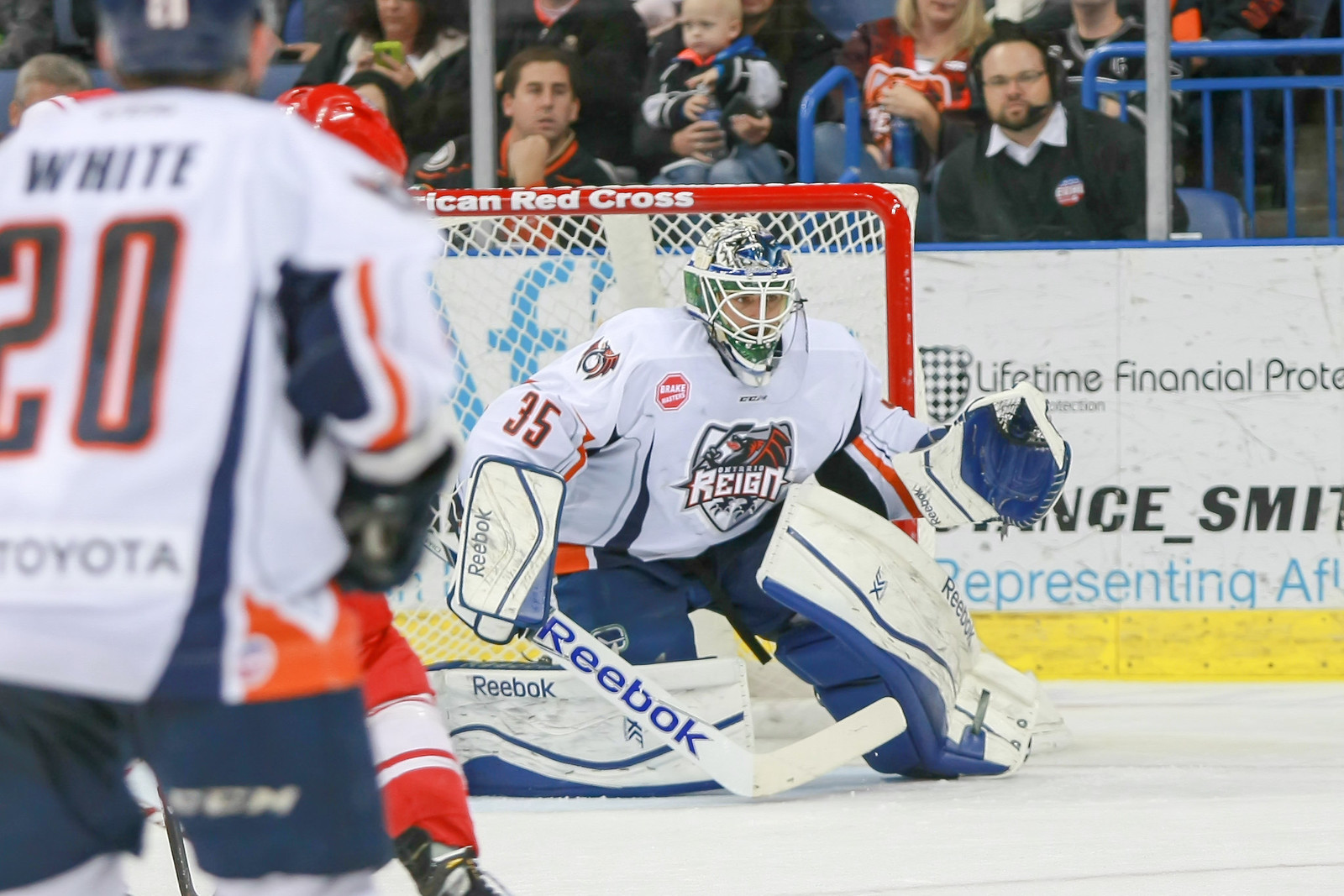The image depicts a live professional hockey game, showcasing a straight-on view of a goalie from the Ontario Reign team, identifiable by his white uniform and Reebok pads and hockey stick. The goalie is poised in front of a net with a red frame and a white net, branded with an American Red Cross advertisement. Behind the glass can be seen a crowd of spectators, including a baby on a parent's lap and a man with headphones, likely a play-by-play announcer. Another player, with the name "White" and the number 20 on the back of his white jersey, is positioned facing the goalie. Advertisements for Lifetime Financial and Aflac adorn the rink, partially visible through the protective glass behind the net. The entire scene plays out on a rink surrounded by white walls and ice, capturing the intense moment of the game.